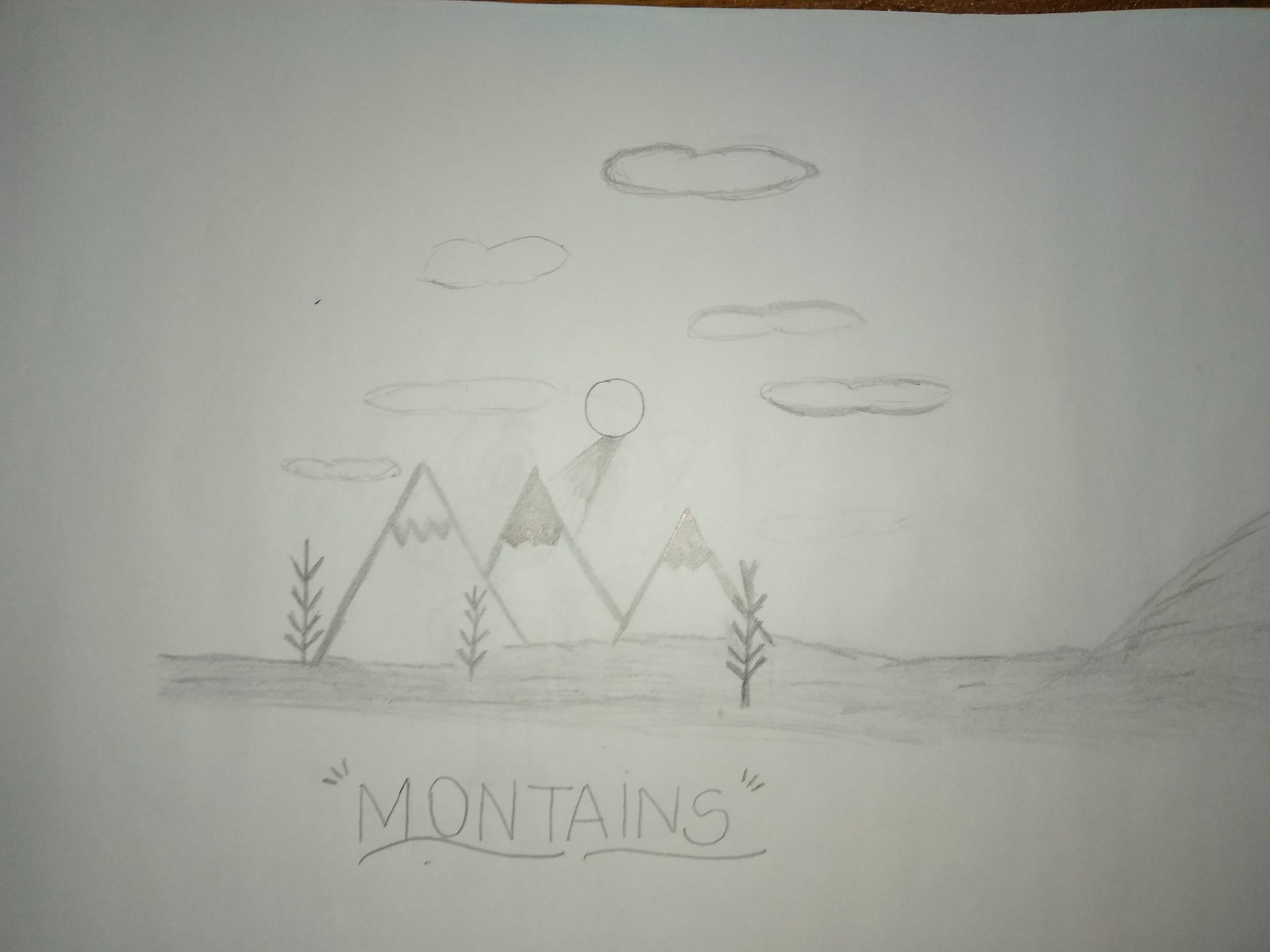In this black-and-white photograph, we observe a child's line drawing executed with black pencil on greyish paper, which might simply appear this way due to poor lighting. Dominating the scene are three sharply pointed mountains at the center, labeled "mountains" at the bottom edge of the drawing. 

The mountains feature zigzag patterns at their peaks, suggesting snow-capped summits, although the central mountain is distinctly shaded in with pencil. Flanking the mountains are small stick-figure trees, grounding the landscape. Further grounding is depicted via a penciled-in terrain around the base of the mountains, with a minor hill present on the far right side of the composition.

Crowning the scene are several thin, oval clouds with heart-shaped centers. Near the top-right quadrant, situated slightly to the right above the central mountain, shines a round circle—likely representing the sun or moon—from which emanate radiating lines, adding a dynamic focal point to the simple yet charming drawing.